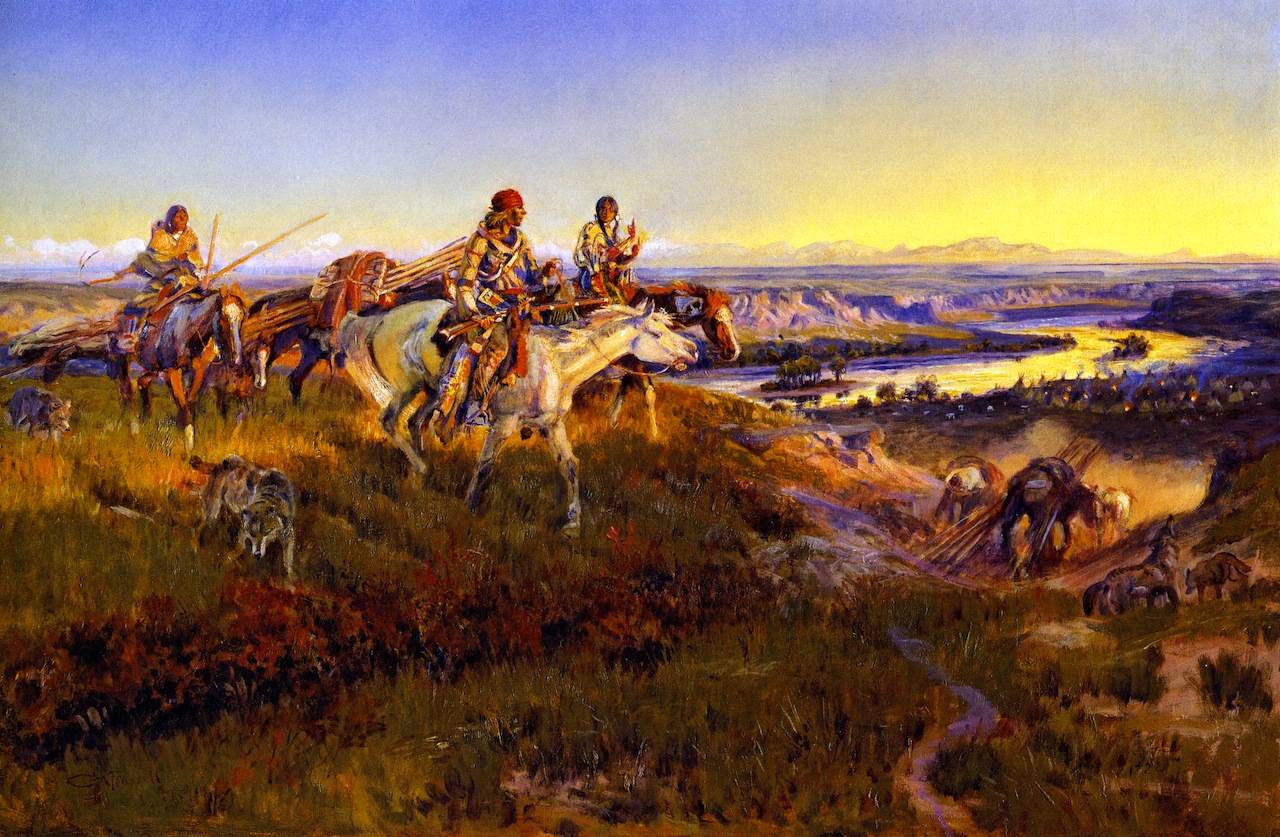This horizontal rectangular painting captures a vibrant and dynamic battlefield scene set in the rough terrain of the southwest, dominated by vivid colors. The central focus is on a hill overlooking a bend in a river, with canyons and mountains in the background. Atop the hill, three figures on horseback—likely Native Americans given their long hair, dress, and adornments—ride purposefully, each holding either a spear, rifle, or stick. The closest rider, mounted on a white horse, is dressed in a striking red, blue, and brown outfit with a red bandana tied around his head and a gun in his hand. Another rider on a brownish horse sports pigtail braids and a blue and tan outfit, with his hands pointed skyward. The third rider on a brown horse holds a stick and a whip, gazing ahead. Accompanying them are canine figures—possibly wolves or dogs—running beside the horses. Behind the riders, additional pack mules or horses can be seen carrying long sticks and packs. A hint of a village with teepees is visible in the background. The scene is meticulously detailed, capturing the rugged beauty of the landscape and the tension of the moment.